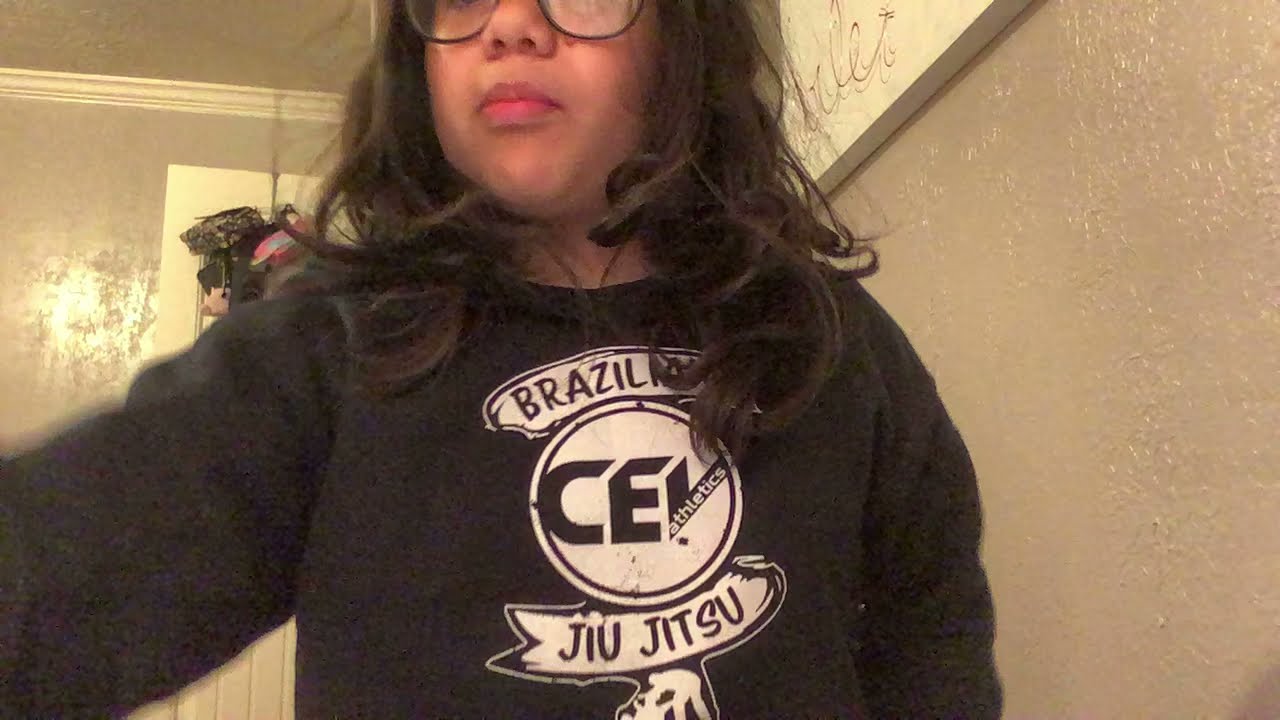This image captures a dark-skinned woman from her torso up to just below her eyes, with the upper part of her head cut off by the frame. She has long, dark hair that is curled at the ends and wears dark black-framed glasses. The background consists of beige walls adorned with paintings. She is dressed in a black sweatshirt with white text that reads "Brazil," encircled by "CEI Athletics," and "Jiu Jitsu" underneath. The woman, who is not smiling, faces slightly to the left, with her arm extended in that direction, and her full lips and cheeks appear more prominent due to the upward-looking angle of the photo.